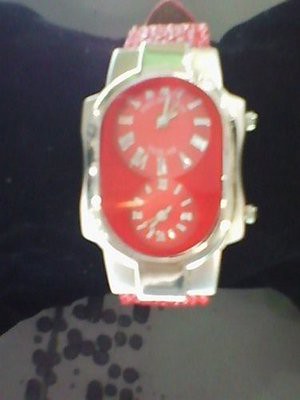A photograph captures an intriguing and modern wristwatch resting on a likely jewelry display pillow made of thick, dark fabric, possibly black. This stylish and unique watch features a band encrusted with small, sparkling gems and colored in a vibrant salmon pink. Dominating the watch is a large, squarish face with a silver frame, partially transparent on the sides, and equipped with two distinct clock faces. The top, slightly larger face displays a time around 2 o'clock, while the bottom one shows approximately 7:40, both using Roman numerals with silver hands and white lettering. The face plates are hues of red, ranging from candy red to bright pink, accented with green stripes. The watch is set against a backdrop transitioning from dark gray at the center to light gray at the top and bottom, with intricate dark gray dots and designs visible on the lower left portion of the image. The overall composition highlights the watch's bold and unusual design, emphasizing its large, clear buttons on the right side and its modern aesthetic.